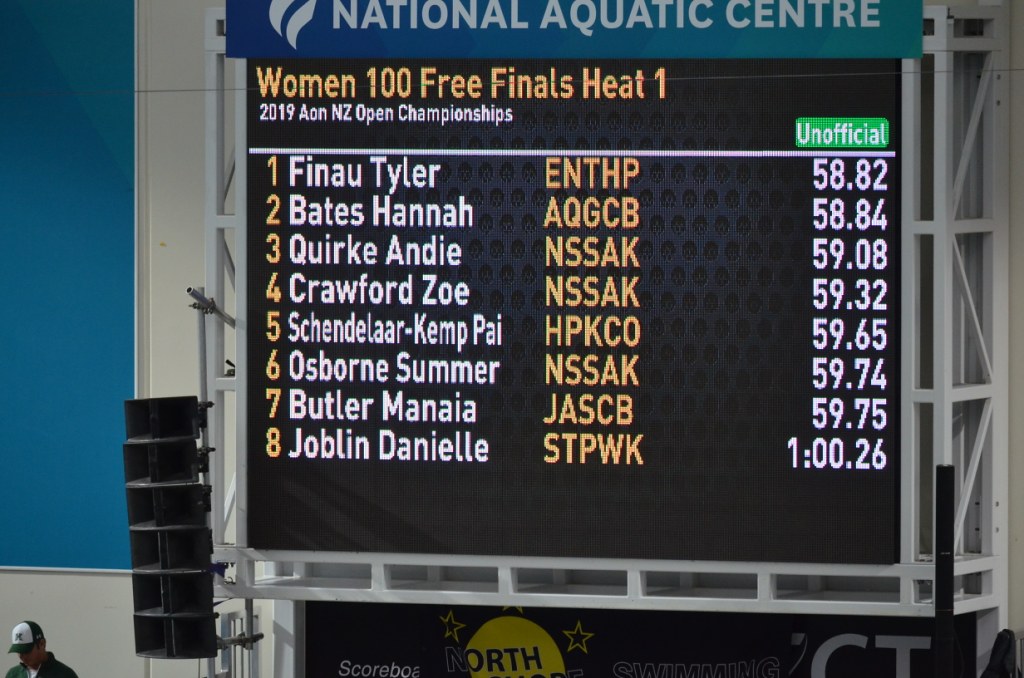This image captures an indoor aquatic center, specifically focusing on a wide rectangular digital scoreboard. The scoreboard, framed in silver metal scaffolding, is central to the image and features a black background adorned with subtle circular patterns. Above the scoreboard, a blue to turquoise gradient banner reads "National Aquatic Center" in white letters. The top line of the digital display indicates "Women 100 Free Finals Heat 1" in yellow letters, followed by "2019 AONNZ Open Championships" in white.

The scoreboard lists eight athletes and their times, indicating it is an unofficial ranking. In first place is Taylor Fennell, with a time of 58.82 seconds, followed closely by Hanna Bates at 58.84 seconds. Andy Quirk is third with 59.08 seconds, and Zoe Crawford is fourth with 59.32 seconds. Fifth place is Chandler Kemp-Pye at 59.65 seconds, Osborne Summer is sixth at 59.74 seconds, Butler Minaya holds seventh at 59.75 seconds, and Danielle Joblin rounds out the list at 1:00.26.

Surrounding the area, there is a white wall on the left with a segment of a bright blue wall visible. A large speaker is mounted on the wall to the right of a person standing in the bottom left corner of the image. Behind the scoreboard, additional blue walls and vertical black speakers are visible, reinforcing the indoor setting of this swimming competition. The overall composition, combined with the listed details and the indoor aquatic setting, indicates this is a photo taken during an athletic event, specifically a swimming championship.